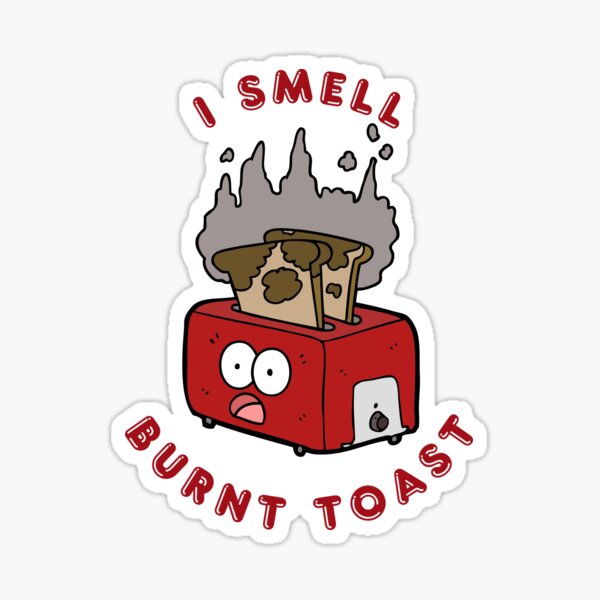This image features a cartoonish, red toaster with a surprised human expression, complete with large white googly eyes and a half-open mouth. The toaster is tilted at an angle and includes a small, silver lever with a black knob on its side. From the top of the toaster, two pieces of bread, characterized by dark and pinkish spots indicative of burning, are popping up. Above the bread, gray smoke swirls, emphasizing the burnt state of the toast. Surrounding the toaster are the words "I smell burnt toast," written in dark red letters. The entire graphic, reminiscent of a sticker or animated illustration, is set against a plain white background, with no additional elements present.